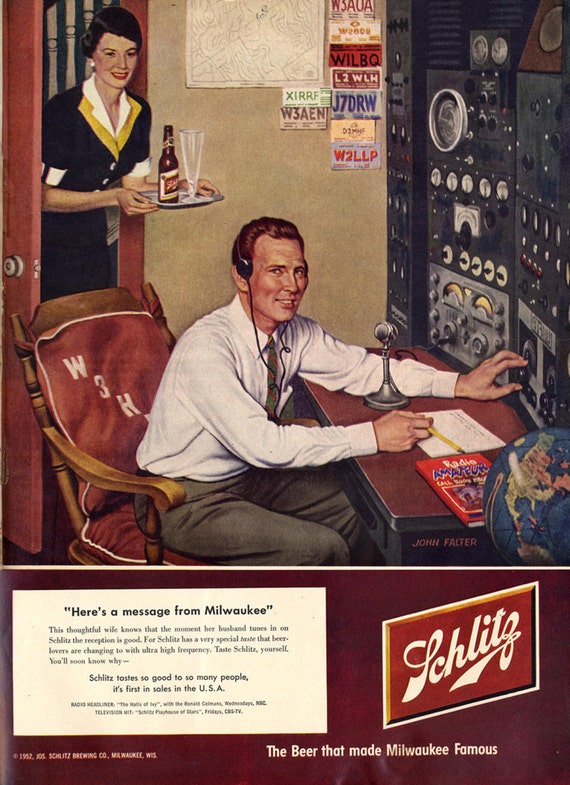The image is a detailed vintage advertisement for Schlitz beer, likely from the 1950s. In the foreground, a man is depicted sitting at a desk, operating a radio station. He wears a white shirt with a tie and gray pants and is positioned in a wooden chair with a red cushion that has "W3H" written on it. The man, smiling and looking at the camera, has a pair of headphones on and holds a pencil in his right hand, while his left hand adjusts a dial on the radio control equipment in front of him. On the desk lies a book titled "Radio Amateur" and a globe.

In the background, a woman dressed in a black dress with white cuffs and a yellow and white collar enters the room carrying a tray. The tray holds a tall Pilsner glass and a bottle of Schlitz beer. The walls of the room are adorned with various license plate-like signs and a roadmap, suggesting it's either a home or a makeshift radio studio.

At the bottom of the poster, it reads: “Here’s a message from Milwaukee. The thoughtful wife knows the moment her husband tunes in on Schlitz, the reception is good. For Schlitz has a very special taste; beer lovers are changing to it with ultra-high frequency. Taste Schlitz yourself—you’ll soon know why it tastes so good to so many people. It’s first in sales in the USA. Schlitz, the beer that made Milwaukee famous.” The Schlitz logo is prominently displayed, and the advertisement underscores the beer's reputed popularity and quality.